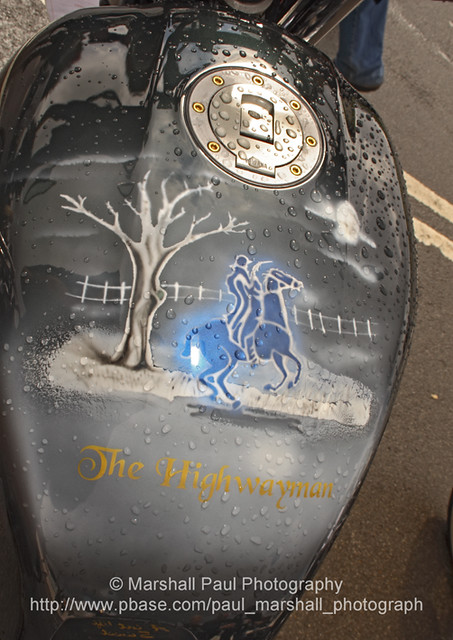The image depicts the top view of a dark forest green motorcycle fuel tank adorned with intricate artwork. Dominating the center is a striking blue horse with a glowing hue, being ridden by a white and blue-clad figure. To the left, a bare tree devoid of leaves nearly taps into a spooky ambiance, augmented by a sketch of a dead tree, a small white and brown leafless tree, and a distant white picket fence under a haunting, overcast sky. In bold yellow letters, somewhat tricky to discern, the tank is emblazoned with the words "The Highwayman." At the top of the tank is a circular silver fuel cap, detailed with little yellow gems, resembling droplets of water or potential raindrops. Completing the scene, beneath the artwork, in white letters, is the mark "© Marshall Paul Photography," accompanied by a website. The entire composition rests on an asphalt road, with visible yellow road stripes providing a sharp contrast against the metallic and painted features of the motorcycle fuel tank.